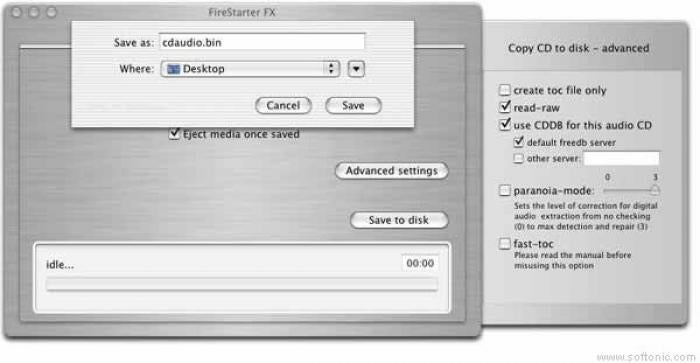The image is a detailed screenshot of the old-fashioned CD burning software FireStarterFX, likely from the late 90s to early 2000s. The interface, reminiscent of older operating systems, features a gray, basic, and dated aesthetic. At the top, the application name "FireStarterFX" is clearly displayed. On the screen, there are two overlapping windows. The first window is titled "Save As," prompting the user to save a CD audio image file to the desktop. Below this, options including "Cancel" and "Save" are visible. The second window, labeled "Copy CD to Disk Advanced," contains several settings with checkboxes. These include options like "Create TOC file," "Read RAW," and "DDB for audio CD," all of which are checked, while "Paranoia mode" and "Fast dot-dash TLC" are also listed, with the latter being unchecked. The software's silver, aluminum-like color scheme adds a nostalgic touch, transporting viewers back to the early days of digital media.